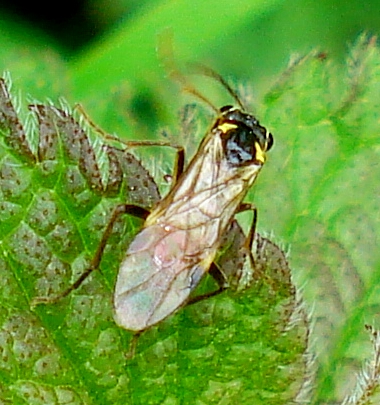This rectangular, near-square nature photograph is a close-up of a winged insect, likely a wasp, perched on a textured, bright green leaf with reddish-brown edges and fine white hairs around the perimeter. The insect has clear, elongated wings that slightly obscure its body, which features a black central stripe flanked by yellow markings. The wasp's long legs and antennae are noticeable, with the antennae seemingly blown to the left, suggesting wind. Its large black eyes are prominently positioned on either side of its head. The background consists of blurred green hues, possibly indicating surrounding trees or branches, giving the image a natural, albeit slightly grainy, and windy impression.